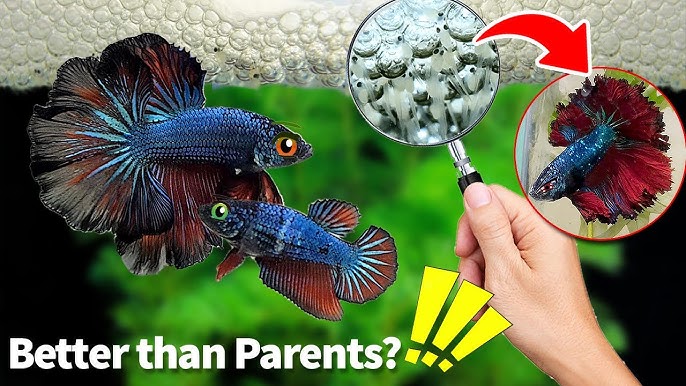The image, reminiscent of a YouTube thumbnail, features a vivid collage of elements. Dominating the left side are two blue betta fish with striking red fins, cut out from a different photograph. The top fish is larger, with orange eyes, while the smaller one below has green eyes. Both have prominent, fan-like fins edged in black. Below the fish is the bold text "Better than parents," styled in white with a question mark and three large yellow exclamation marks. This text has a notable drop shadow effect for emphasis.

The background is an indistinct green and black blur, suggesting vegetation but remaining out of focus. On the right, a hand holds a magnifying glass that enlarges some white, frothy bubbles near the top of the image. Within the magnified view, tiny, transparent baby fish are visible. A red arrow emerges from the magnified area, pointing towards a red circle on the right side of the image. Inside this circle, another blue betta fish with vivid fins, similar to those on the left, is displayed. The entire composition appears to be a composite image assembled using Photoshop techniques.